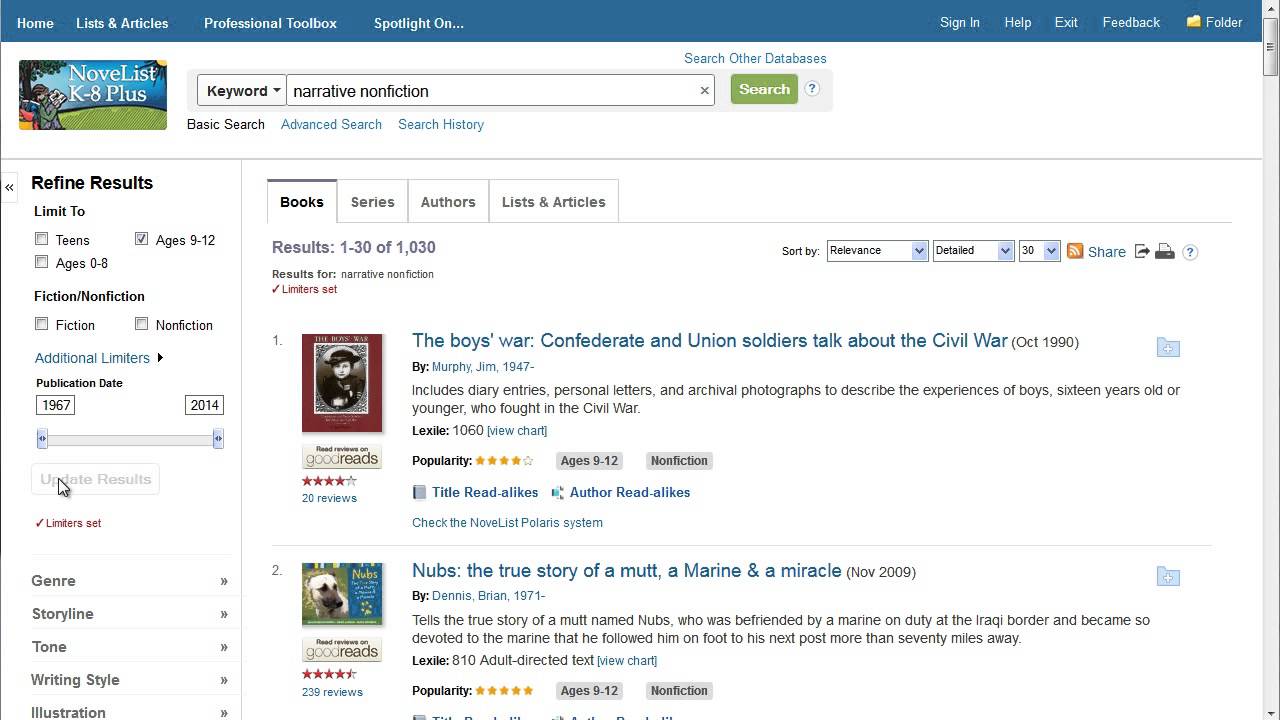**Caption:**

The webpage displayed on a computer screen showcases a specialized store interface for books, particularly geared towards children from kindergarten through eighth grade. The top of the screen features a blue navigation bar. On the left side, it includes options labeled Home, Lists and Articles, Professional Toolbox, and Spotlight On. On the right side, the bar offers Sign In, Help, Exit, Feedback, and Folder options.

Below this navigation bar, the main content area of the page is predominantly white. A small icon indicating "Novelist K-8+" suggests that the site focuses on providing literary resources for young readers. There is a search function available, allowing users to search by keyword with a drop-down menu and text input labeled "Narrative Nonfiction." A search button is also present, accompanied by options to explore other databases with Basic Search, Advanced Search, and Search History functionalities.

Directly below the search options, a segmented area displays further refinement options. Users can limit results to age groups 9 through 12, or 0 through 8, with checkboxes for fiction and nonfiction categories. Additional filters include publication dates (adjustable from 1967 to 2014) and other criteria such as genre, storyline, tone, writing style, or illustrations.

The current search results display two books: "The Boys' War: Confederate and Union Soldiers" and "NUBS: The True Story of a Mutt, a Marine, and a Miracle." Users can view more details and organize results by book, series, author, and lists and articles.